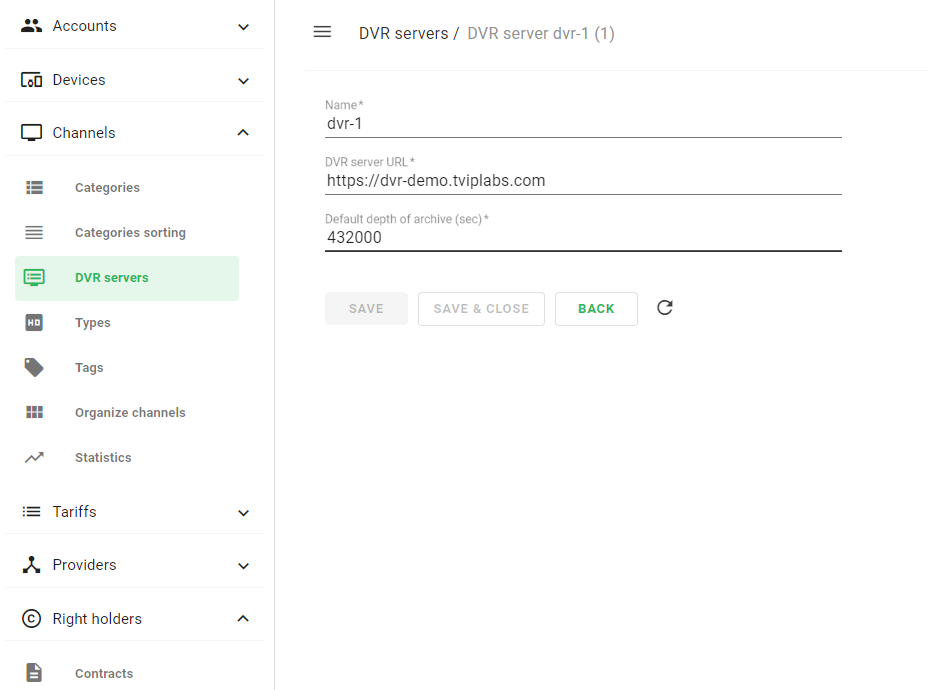The image depicts the interface of an Android device, featuring a detailed and organized settings menu for managing various system aspects. 

On the left side of the screen, there's a categorized list that includes: 
- Accounts 
- Devices 
- Channels 
- Categories 
- Category Sorting 
- DVR Service 
- Types 
- Tags 
- Organized Channels 
- Statistics 
- Tariffs 
- Providers 
- Right Holders 
- Contracts

Each entry in this list has its own unique order and is organized under specific folders and categories.

To the right side of the screen, the "DVR Service" option is selected, highlighted with a green, semi-translucent overlay. This section provides more detailed information and settings related to DVR services. At the top left corner of this section, a hamburger menu icon is visible, followed by the title, which reads: "DVR Service / DVR Service DVR-1 (1)".

Below the title, there is a form containing three elements:
1. **Name**: The input field is filled with "DVR".
2. **DVR Server URL**: The input field contains a URL starting with "https://".
3. **Default Depth of Archive**: This is labeled "SEC" (likely denoting seconds), with "432000" specified as its value.

Underneath the form, there are three buttons. The "Save" and "Save and Close" buttons are both grayed out, indicating they are not currently active or clickable. The "Back" button is active, displayed with green text. Next to the back button is a refresh icon.